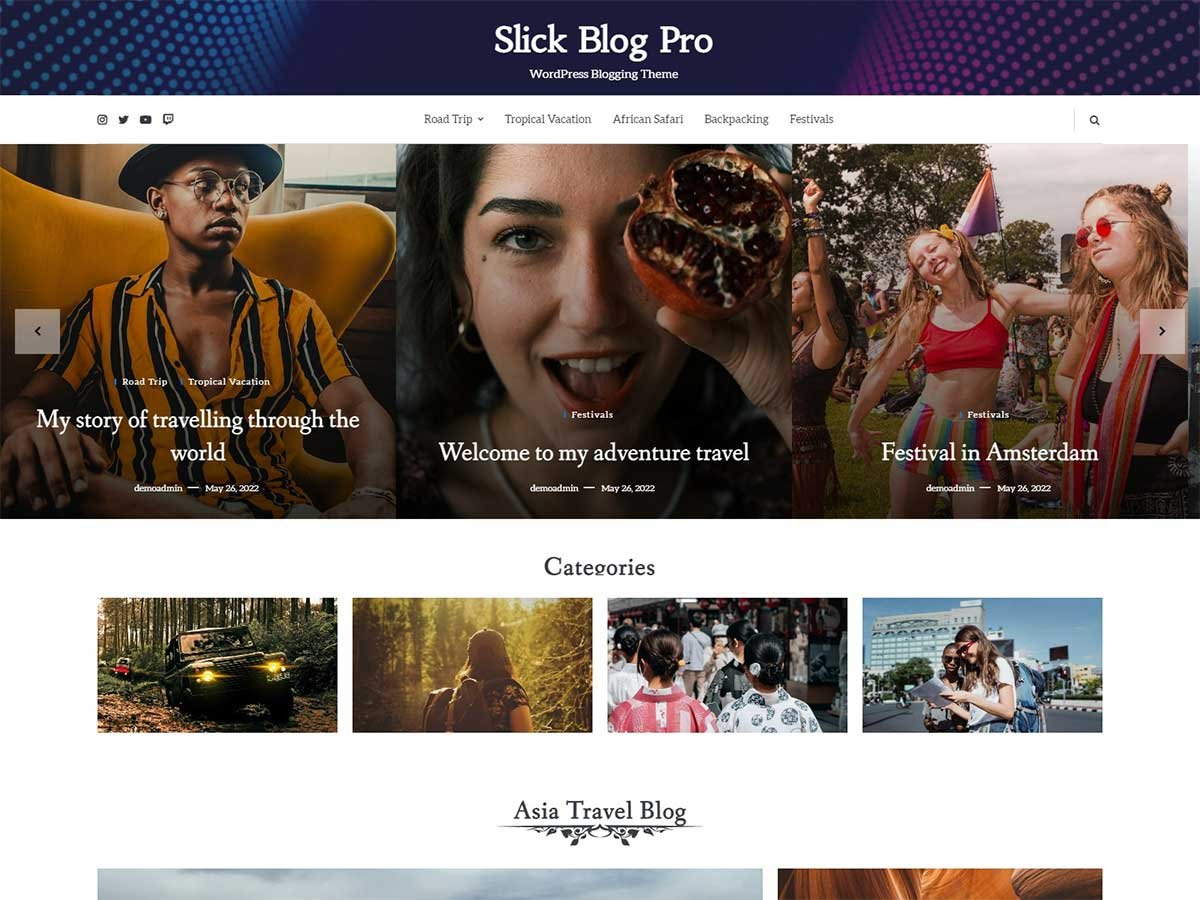The image features a sleek design with a blue and purple border at the top, adorned with geometric patterns. The center background is dark blue, prominently displaying white text that reads "Slick Blog Pro, WordPress Blogging Theme." Below this, a menu in blurry text lists various categories including "Road Trip," "Tropical Vacation," "African Safari," "Backpacking," and "Festivals." 

The content below the menu showcases three images. On the left, there's a photograph of a man with dark skin, wearing a yellow shirt with black and white vertical stripes, glasses, and a wide-brim hat. The caption reads, "My Story of Traveling Through the World." 

To the right, a woman is seen holding a halved pomegranate close to the camera, accompanied by the text, "Festivals, Welcome to My Adventure Travel."